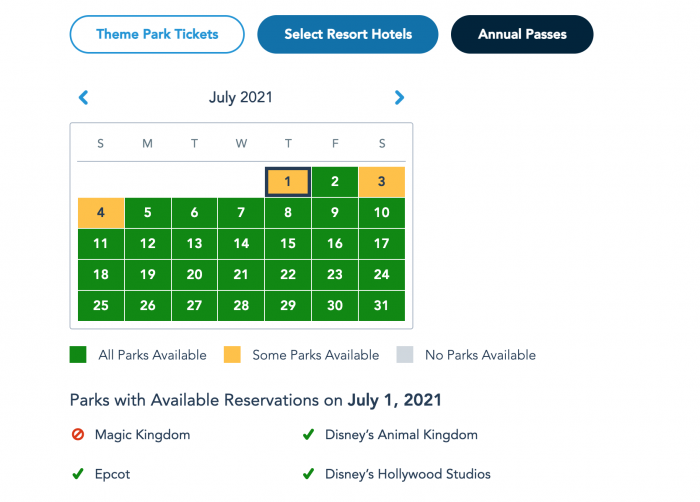A detailed schedule for planning trips to Disney theme parks, this image showcases a July 2021 calendar. Highlighted in various colors according to availability, nearly all dates are marked in green for “All Parks Available.” Exceptions are notable: July 1st, July 3rd, and July 4th are marked in yellow for “Some Parks Available,” and no dates are indicated in gray for “No Parks Available.” A color code below the calendar provides a key to these markings.

Below the color code, details about park availability on July 1st, 2021, are provided. The screen indicates that while Magic Kingdom is not available on that date (signified by a red circle with a line through it), Epcot, Disney's Animal Kingdom, and Disney's Hollywood Studios are all available (indicated by green check marks).

At the very top of the page, users can see three menu categories: Theme Park Tickets, Select Resort Hotels, and Annual Passes, emphasizing the page's focus on reservations for Disney theme parks and associated accommodations.